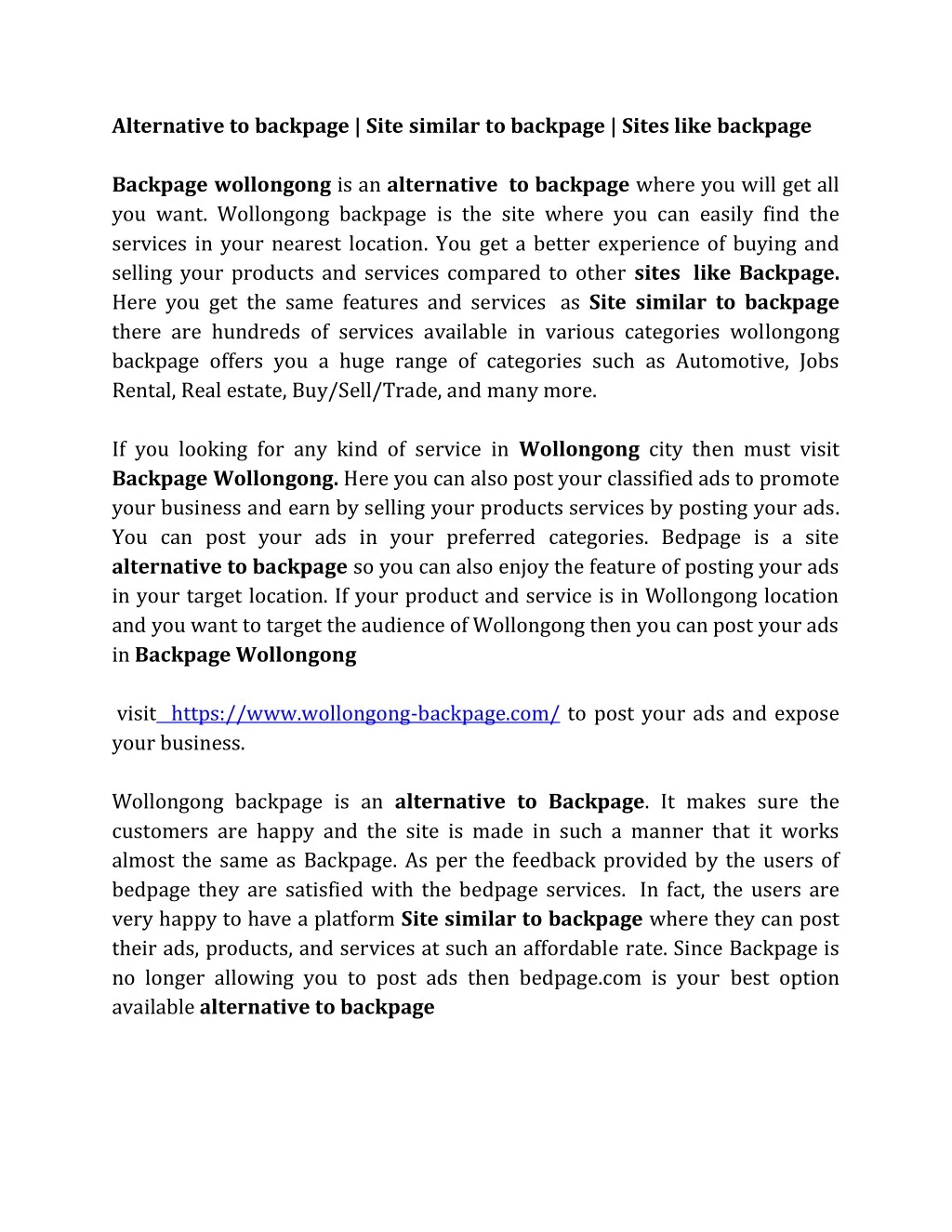The image shows a simple, white-background page filled with black text focusing on alternatives to Backpage. At the top, bold text repeatedly states "Alternative to Backpage," "Sites similar to Backpage," and "Sites like Backpage." The body text, organized into four paragraphs, describes Wallangong Backpage as a comprehensive alternative platform where users can buy and sell products and services. The site offers categories comparable to Backpage, including automotive, jobs, rentals, real estate, and more. Detailed instructions and features of Wallangong Backpage are outlined, emphasizing its user-friendly experience. A website link, www.walagongbackpage.com, is included in the third paragraph for posting ads and promoting businesses.